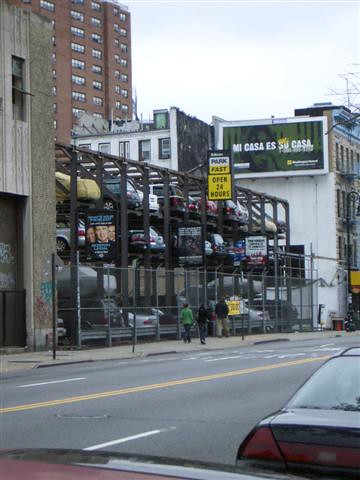The photograph appears to be from the 1970s or 80s, capturing a bleak urban scene dominated by muted grays and dark colors. In the background to the top left, an imposing, very tall tenement building suggests a densely populated area. In front of the tenement, an iron girder structure resembling a multi-level marina storage facility for boats is repurposed to hold cars, rising three stories high with no walls. A towering chain-link fence topped with barbed wire partially obscures this structure, leading to an entrance reminiscent of a parking garage. The foreground reveals a street marked by a yellow center line and white lane dividers. Two cars are parked side by side, and three individuals can be seen: two walking and one sitting. The scene evokes a sense of urban decay and desolation.